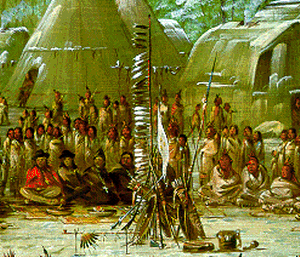This is a detailed, artistic portrayal of a gathering of Native Americans in a circle, possibly indicating an important meeting or ceremony. The image, likely from an old drawing or print of a painting, exudes a greenish-yellow hue and contains white brushstroke highlights that add to its artistic feel. In the foreground, a central arrangement of long poles adorned with feathers, spears, and arrows takes focus, suggesting the preparation or conclusion of a ritual. Surrounding this central pole, Native American figures wrapped in white cloaks or blankets sit, indicating the season might be cold. Some are seated in rows, while others stand in the background, all donning traditional headbands and feathered headdresses. The upper portion of the image features several large tipi structures. Additionally, there are figures that might be mistaken for pilgrims or priests with distinctive hats and robes, seated at the front with plates and mats before them, indicating a possible interaction between different cultural groups or differing attire within the tribe itself. The small, square nature of the image, along with its artistic rendering, restricts the visibility of finer details.